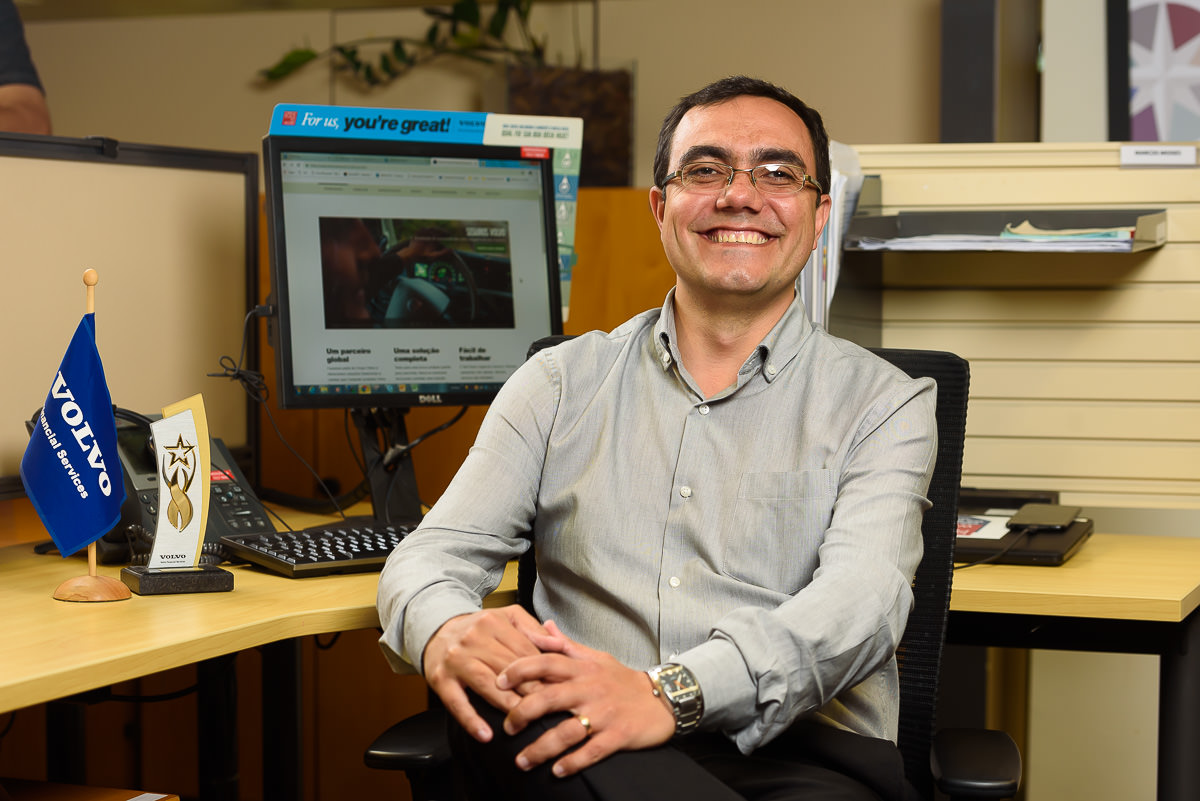A professionally-done photograph features a smiling Caucasian man sitting in a black office chair at a light brown wooden corner desk, characterized by its short, attached walls. The man, who may be a CEO or a high-ranking professional, is dressed in a gray button-up shirt with white buttons, tucked into black dress pants. The top collar button is undone and the shirt features a front chest pocket. He wears a silver wristwatch on his left wrist and a gold wedding ring on his left ring finger. His short brown hair and dark-colored glasses frame his smiling face. Behind him, the beige office partitions are adorned with work trays. On his desk, a laptop screen displays an article about cars with the headline, "For Us, You're Great," and is accompanied by a Volvo sticker. To his right, multiple tabs are open on a web browser, and two award trophies from Volvo are prominently displayed, indicating a professional association with Volvo Commercial Services.